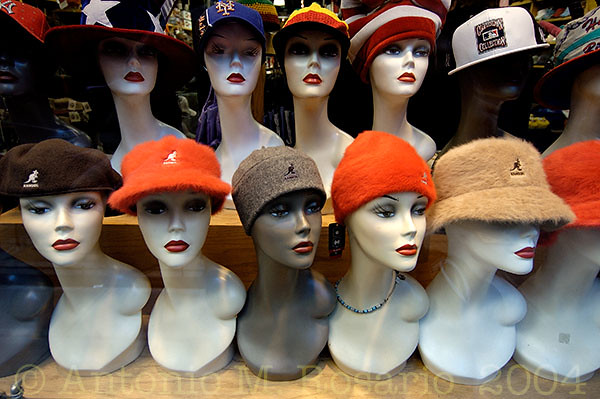This photograph captures a detailed display of mannequin heads adorned with various hats, typically found in a retail store setting. The display consists of two rows, each featuring six mannequin heads. The bottom row predominantly showcases Kangol caps, identifiable by the distinctive kangaroo logo, in assorted colors like brown, white, and fluffy orange. The top row features a diverse array of hats including a USA baseball cap, a New York Mets cap, a red and yellow cap, a Rastafarian beanie, a red and white stocking cap reminiscent of a Santa hat, and a tan bucket hat. The mannequins, primarily Caucasian-looking, with slender faces and noses, have flat chests without any defined busts. There is a singular mannequin with a brown-colored skin tone among them. Displayed on a wooden case, the mannequins, mostly facing forward or slightly to the right, exude a sense of uniformity, underlined by the watermark "Antonio M. Rosario, 2004" at the bottom of the photo, further affirming its authenticity and vintage appeal.